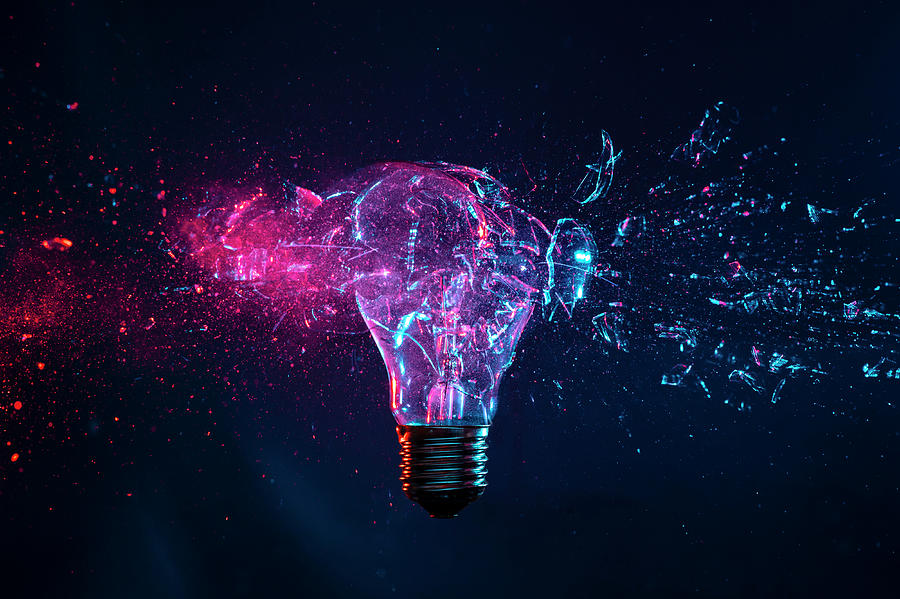This detailed image presents a glass light bulb caught mid-explosion, creating a mesmerizing, almost surreal scene. The light bulb, positioned at the center of the frame, is shattering dramatically, with pieces of glass scattering in all directions. The left side of the bulb is tinged with a vibrant pinkish hue, while the right side is predominantly blue, interspersed with specks of pink and purple. Even amid the explosion, the bulb emits a fluorescent glow, accentuating the scattered fragments with shades of pink, purple, and blue. The background features a deep, almost black, blue, providing a stark contrast that highlights the luminosity of the shattered glass. The composition, while simple, evokes an abstract artwork, capturing the fleeting moment of destruction in exquisite detail, as though a bullet or some unseen force has just passed through, leaving a burst of color and light in its wake.